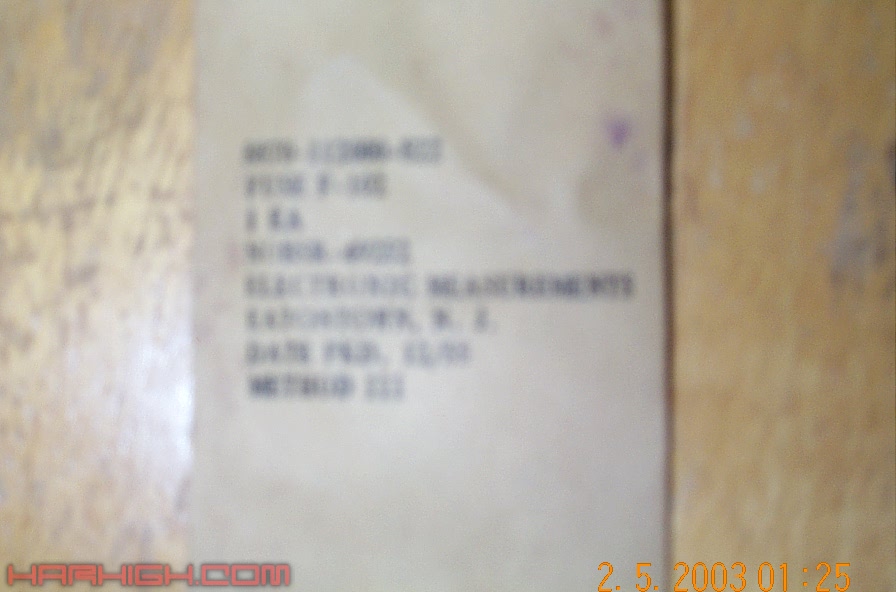A highly out-of-focus image featuring a blurred beige background and a white till receipt centrally positioned. A light source shines from the left-hand side, casting a subtle illumination across the scene. The lower edge of the receipt displays indistinct red lettering, with the text rendered unreadable and its language unidentifiable. At the bottom right corner of the image, a sequence of yellow numbers is visible, extending from the receipt onto the surrounding background. Due to the significant blurriness, the details on the receipt, including any printed content, cannot be deciphered.